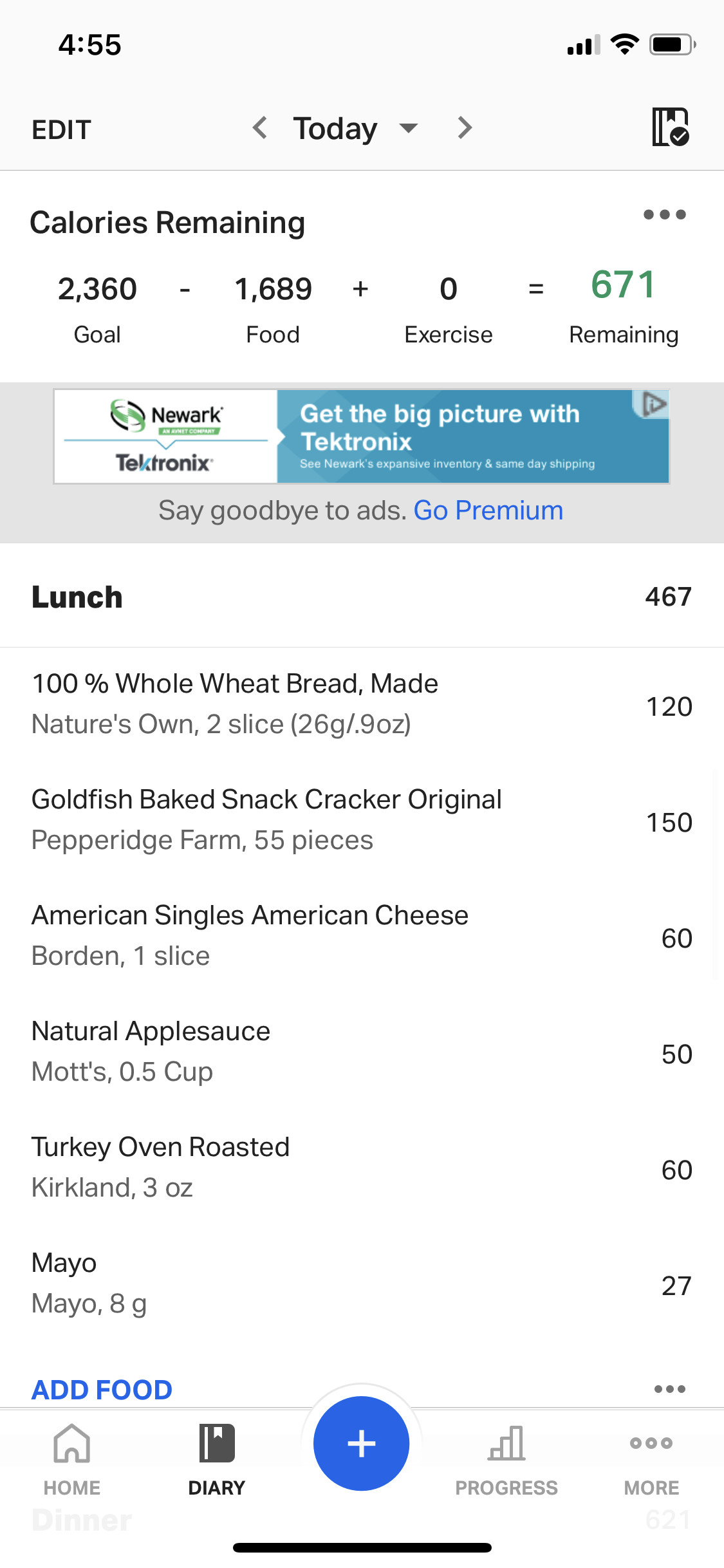A smartphone screen displaying a calorie tracking app interface at 4:55 PM. The app summarizes the user's daily calorie intake goal set at 2,360 calories. After accounting for consumed food (1,689 calories) and no exercise, the user has 671 calories remaining for the day. Focused prominently on the screen is the lunch section, detailing a meal totaling 467 calories. The breakdown of the lunch includes 120 calories from 100% whole wheat bread, 150 calories from Goldfish Baked Snack Crackers, 60 calories from an American single slice of cheese, 50 calories from natural applesauce, 60 calories from oven-roasted turkey, and 27 calories from mayonnaise. Below the meal summary, an advertisement for New York Tektronik prompts users to “Get the big picture with Tektronik,” with an option to go premium and remove ads for an uninterrupted app experience.